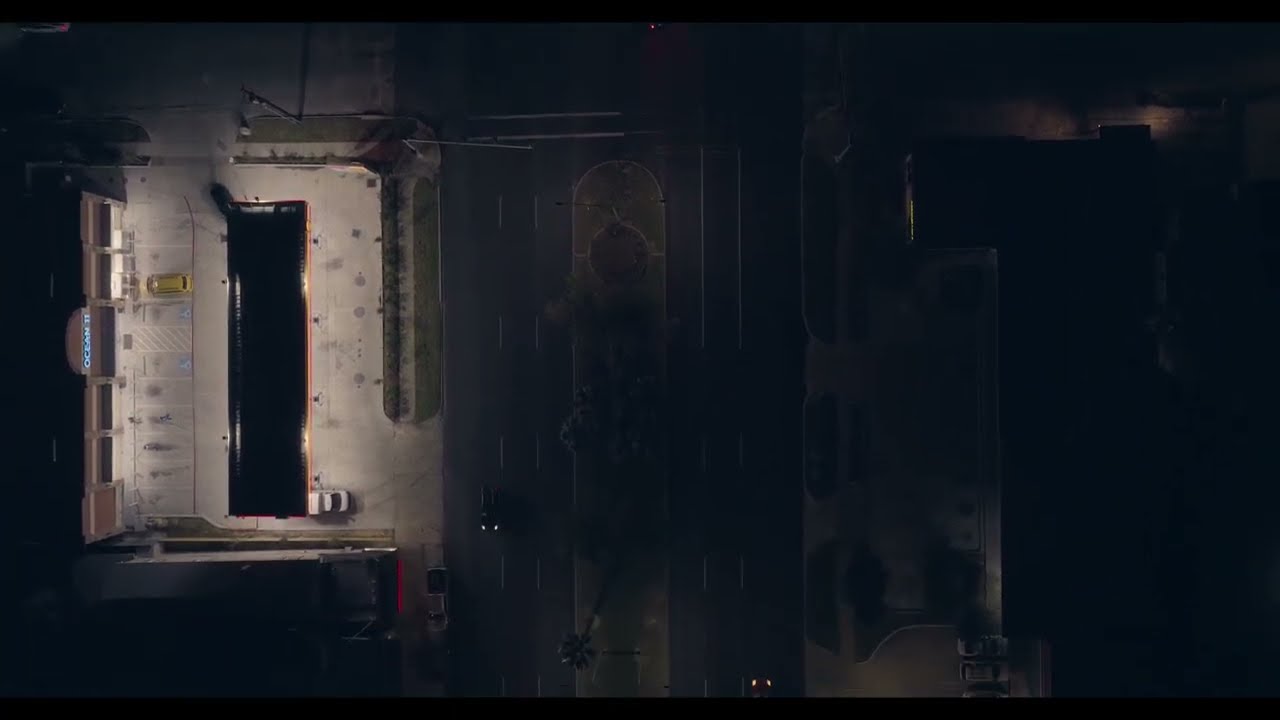This horizontal rectangular image, framed by black borders at the top and bottom, captures an overhead nighttime view of a street scene with sparse lighting. To the left, an illuminated area reveals a parking lot with a yellow car and a white car, adjacent to a building or sign that reads "Ocean 11" in blue lit-up letters. The scene is very dark, indicative of night, and details fade as you look toward the center and right side of the image. Two roads with dashed white lines and a central median intersect the area, with cars' headlights visible traveling in both directions. On the far right, a small section of another parking lot can be discerned at the bottom, showing three cars parked next to each other. The overall atmosphere is industrial and moody, with the focus drawn to the lit parking lot and the "Ocean 11" signage against the dark surroundings.